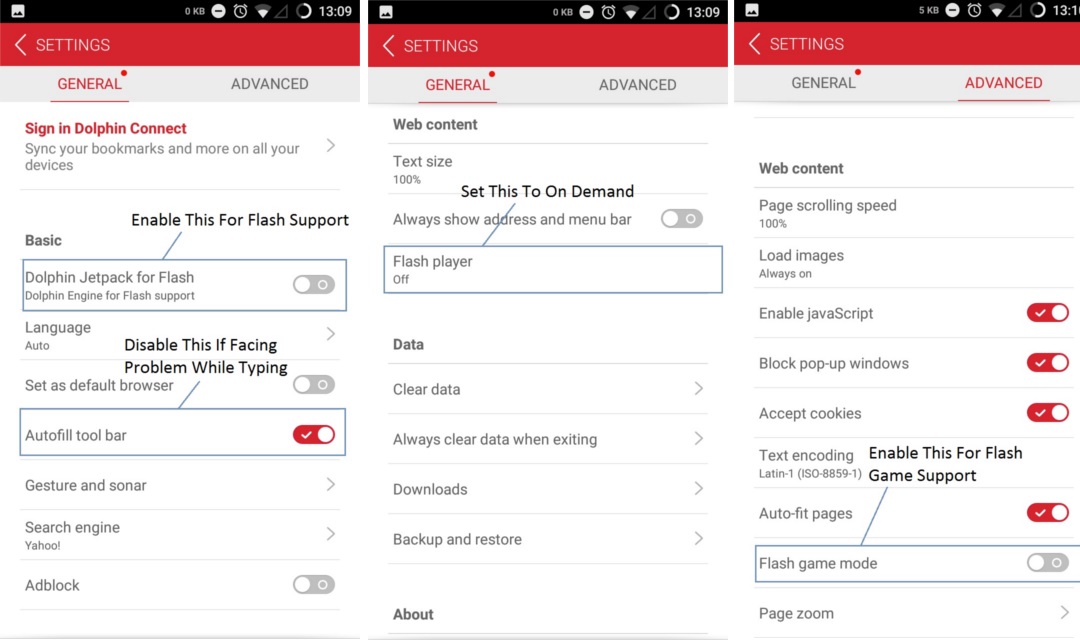The image comprises three smartphone screenshots, all from the same website, indicated by the consistent color scheme. Each screenshot features a black header at the top, just beneath which lies a vibrant red section labeled "Settings." In this red section, tabs labeled "General" and "Advanced" are visible.

Below the red header, the main content is displayed against a light gray background transitioning into white. The screenshot on the right particularly details web content settings. Under gray-colored text "Web Content," there is a setting titled "Page Scrolling Speed" marked at 100%. Additional options include "Load Images" and "Enable JavaScript," both of which have been activated, as indicated by red radio buttons with white checkmarks. Similarly, "Block Pop-up Windows" and "Accept Cookies" settings are enabled. Further down, the option "Text Encoding" appears, followed by a bold, black statement: "Enable this for Flash game support."

The other two screenshots portray different settings but maintain the same layout and design, emphasizing the website's uniform interface for adjusting various preferences.